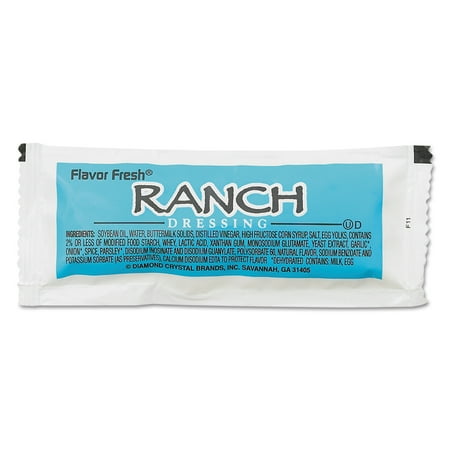The image depicts an upright packet of ranch dressing often found in restaurants or takeaways. The packet is predominantly white with perforated edges for easy tearing and a few black details at the corners. A light blue label occupies much of the packet, featuring "Flavor Fresh ®" in the top left corner. Below, in all caps and black font with a white border, the word "RANCH" is prominently displayed, followed by "dressing" in white, framed by black lines on either side. 

The ingredients list is detailed in bold and regular sans serif fonts, listing soybean oil, water, buttermilk solids, distilled vinegar, high fructose corn syrup, egg yolks, among other components. Notably, dietary symbols appear beside the ingredient list. At the bottom, the allergen information states "Contains: milk, egg." The manufacturer's details, "Diamond Crystal Brands, Inc. Savannah, Georgia 31405," are printed in bold all caps at the bottom center. The packet is photographed against a white background, suggesting it's possibly from a store page for catering businesses.